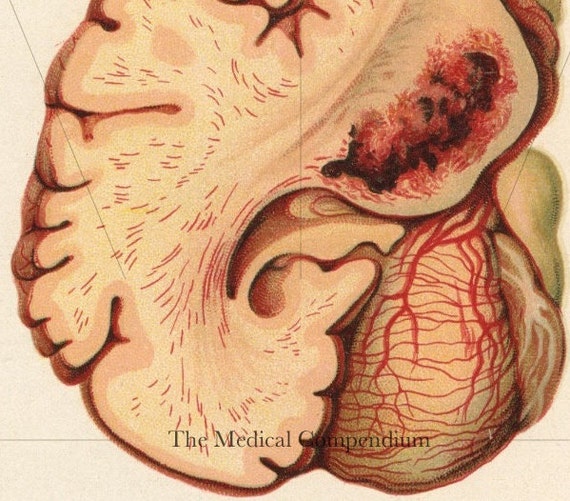The image is a detailed, vintage representation of a sliced brain, labeled at the bottom as "The Medical Compendium." This colorful illustration ranges in hues from peach, tan, red, to light pink and beige, with some black areas, capturing the intricate details of blood vessels and areas of apparent abnormalities. Despite its clear and well-lit presentation, it's not an actual photograph but rather an illustrated depiction. There is a noticeable heart depicted on the lower right side of the image, showing veins and muscular structures, suggesting a further exploration of anatomical detailing. This might indicate various medical conditions affecting the brain, with some areas looking diseased and inflamed.